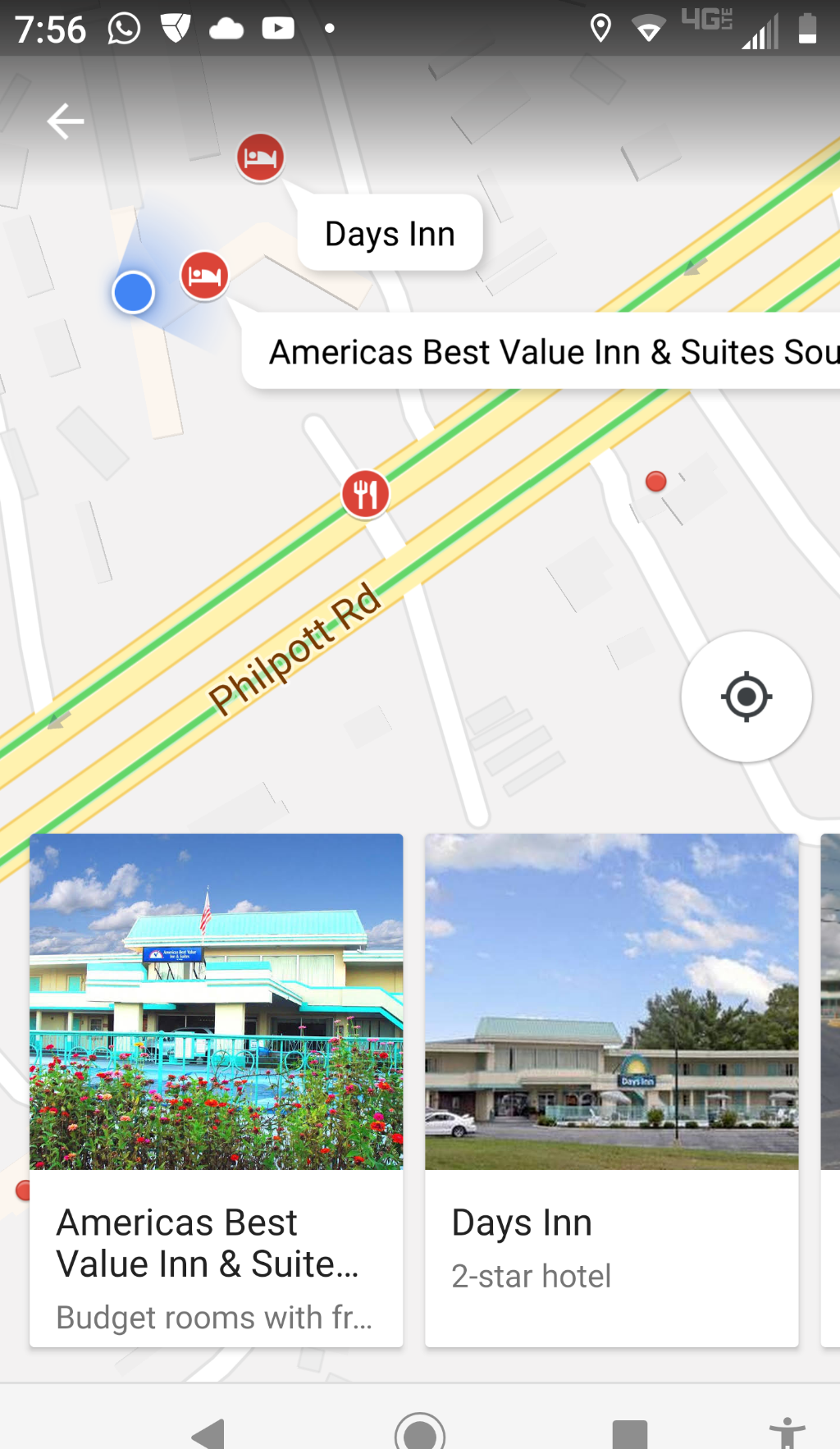The image depicts a screenshot of a map interface, likely from a hotel search application. The map itself shows various geographical elements and includes markers for several hotels. Notably, there are visible markers for a Days Inn and an America's Best Value Inn. The user's current location is indicated by a blue dot, suggesting that they are in close proximity to these hotels and actively searching for accommodations.

Two roads, Philpot Road and another unnamed road, are visible on the map, providing orientation and access points to the highlighted hotels. Additionally, a dining establishment is marked nearby, offering viewers an indication of local amenities.

At the bottom of the image, there are thumbnail photographs providing a preview of the hotels. The America's Best Value Inn is featured with an image showcasing its older architectural style, painted in turquoise and white, complemented by an array of vibrant flowers in front of the building. The Days Inn, rated as a two-star motel, appears to have an even more dated exterior, adhering to a traditional motel layout.

There are also visible control buttons at the bottom of the screen, which likely offer additional options for navigating the map or adjusting the search parameters.